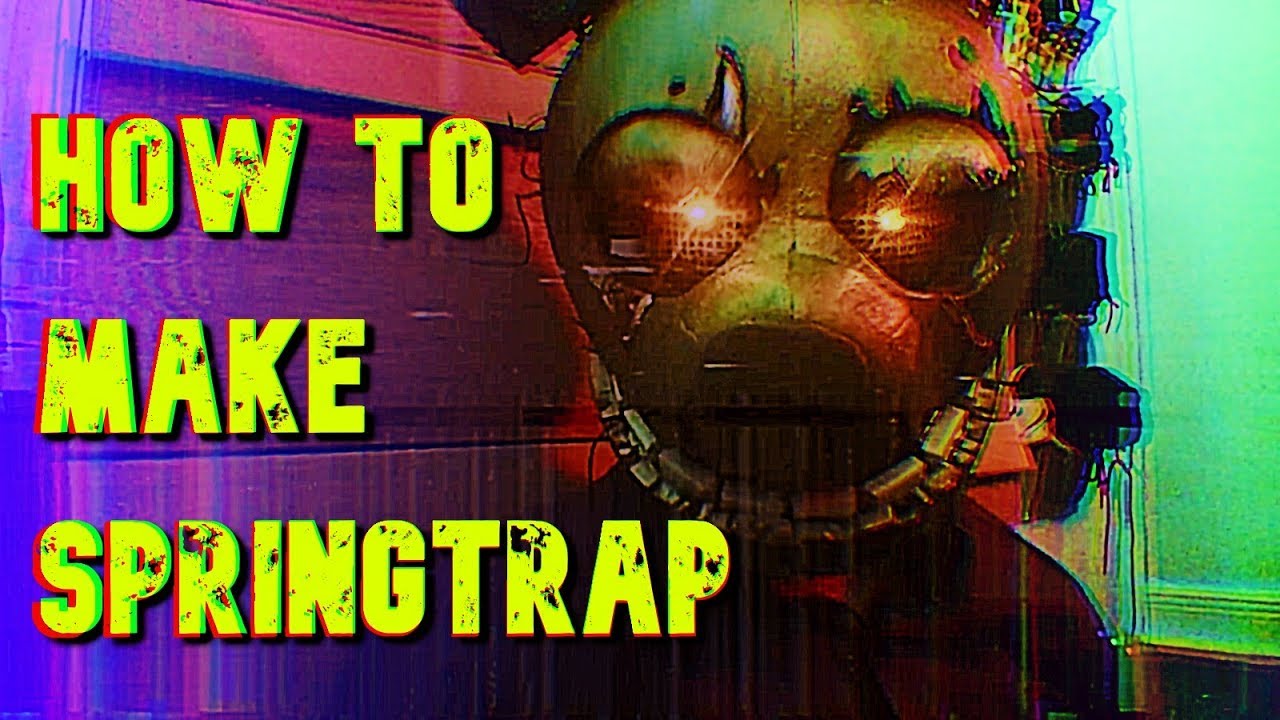The image depicts an individual or creature wearing a large, metal mask with distinctive, oversized bug eyes that reflect white light and a small respirator mouth vent. Chains hang around the neck of the mask, which is beige and tan in color. The background transitions through cyan, purple, violet, and pink, resembling a neon color-changing sign. A retro filter overlays the entire scene, adding to its abstract and nostalgic feel. Dominating the image is a large text overlay in big, yellow capital letters with black splotches resembling rust, reading "HOW TO MAKE SPRINGTRAP."